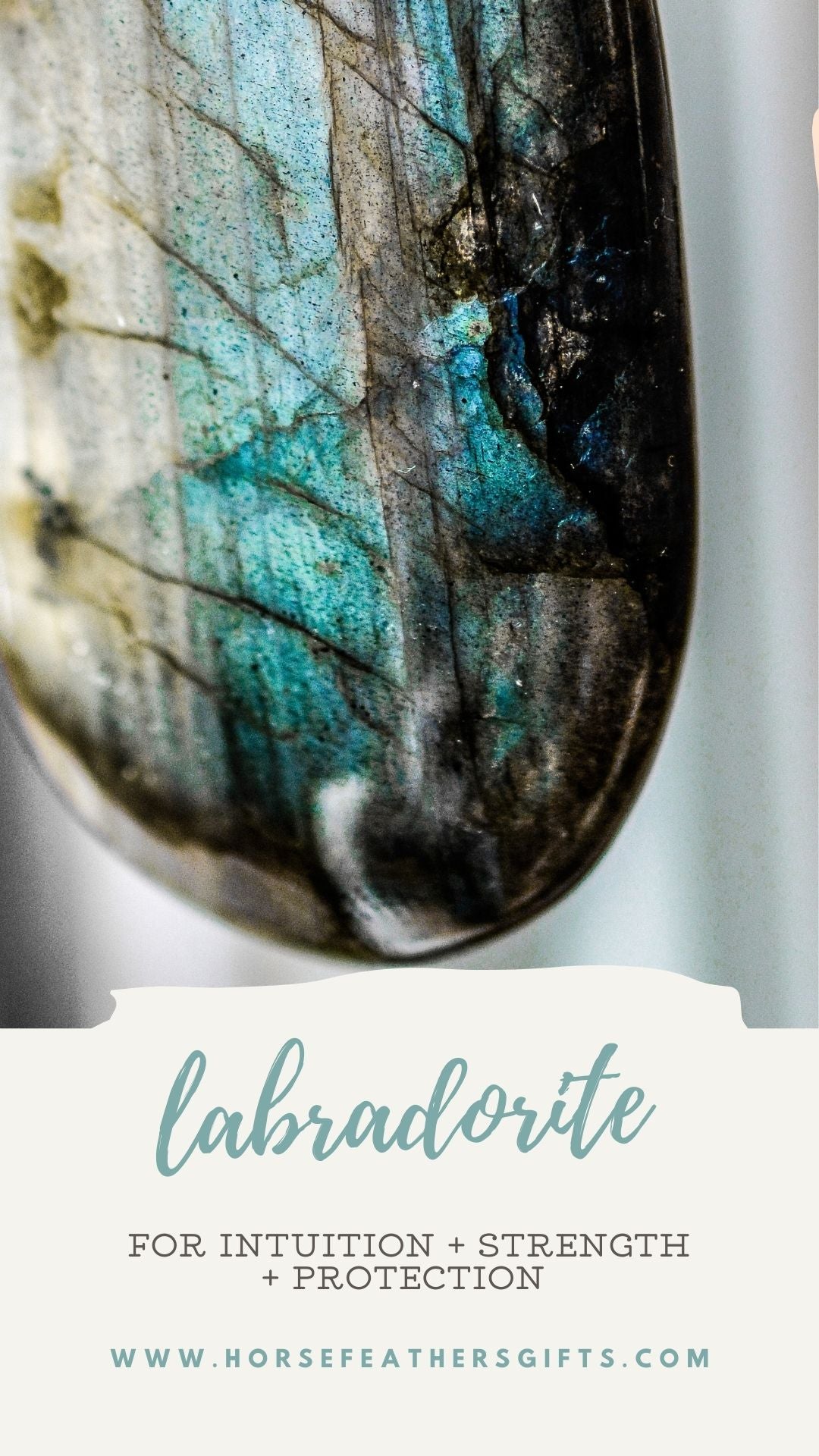The image is a promotional graphic for a business featuring a detailed photograph of a Labradorite stone. The top portion of the image showcases a close-up of the stone's elongated head, which faces downward and occupies most of the image. The stone’s coloration primarily includes hues of blue with dark black at the edges and a mixture of grayish-green, white, and brown lines and cracks. The eye of the stone is prominently visible, contributing to its mystique. The bottom third of the image is a gray banner with an uneven edge that contains multiple lines of text. Written in cursive blue font, the word "Labradorite" stands out, followed by the phrase "for intuition plus strength plus protection" in black print. Below this, the business's URL, "www.horsefeathersgifts.com," is displayed in blue capitals. This promotional flyer effectively combines the striking visual of the Labradorite stone with its associated qualities and the business information.